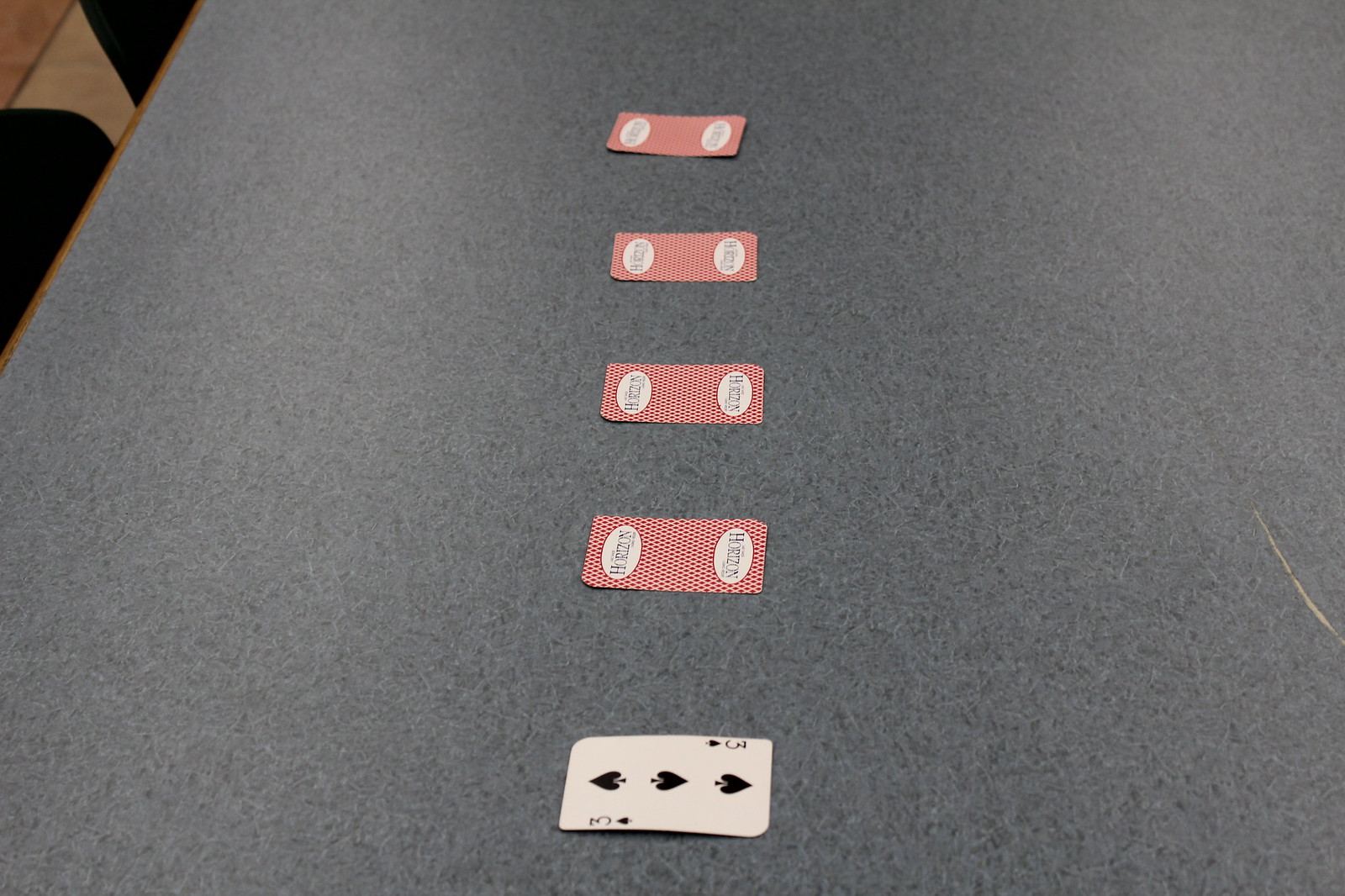The image appears to be taken in a game room or a casino, specifically around a table used for playing card games. The table in the center has a distinctive blue surface with a wooden edge bordering it. There are five cards arranged on the table: four are face down, featuring red backs with an unreadable word inside oval shapes on both ends; the fifth card is face up and reveals the three of spades. Two chairs are neatly pushed into the table, suggesting recent or upcoming use. The visible portion of the floor appears to be made of wood or laminate. Notably, the right side of the table displays a significant scratch, revealing an unattractive white or wooden color beneath the blue surface, indicating extensive wear and tear.